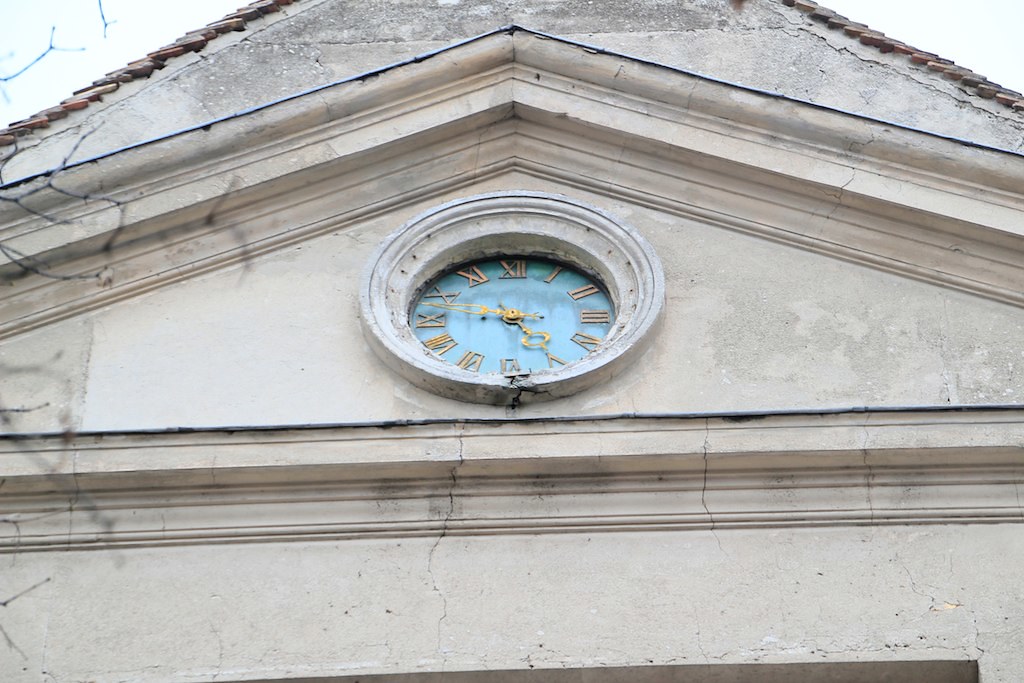A photograph captures a weathered building showing signs of age with visible cracks marring its facade. Prominently featured just below the roof's peak is a classic clock displaying Roman numerals in a golden or brass hue, matching the color of its hands. The clock's background is a light blue, contrasting with the worn textures of the building. Architectural elements frame the clock, enhancing its prominence. The photograph is cropped just below the roof’s apex, revealing only a portion of the building's peak.